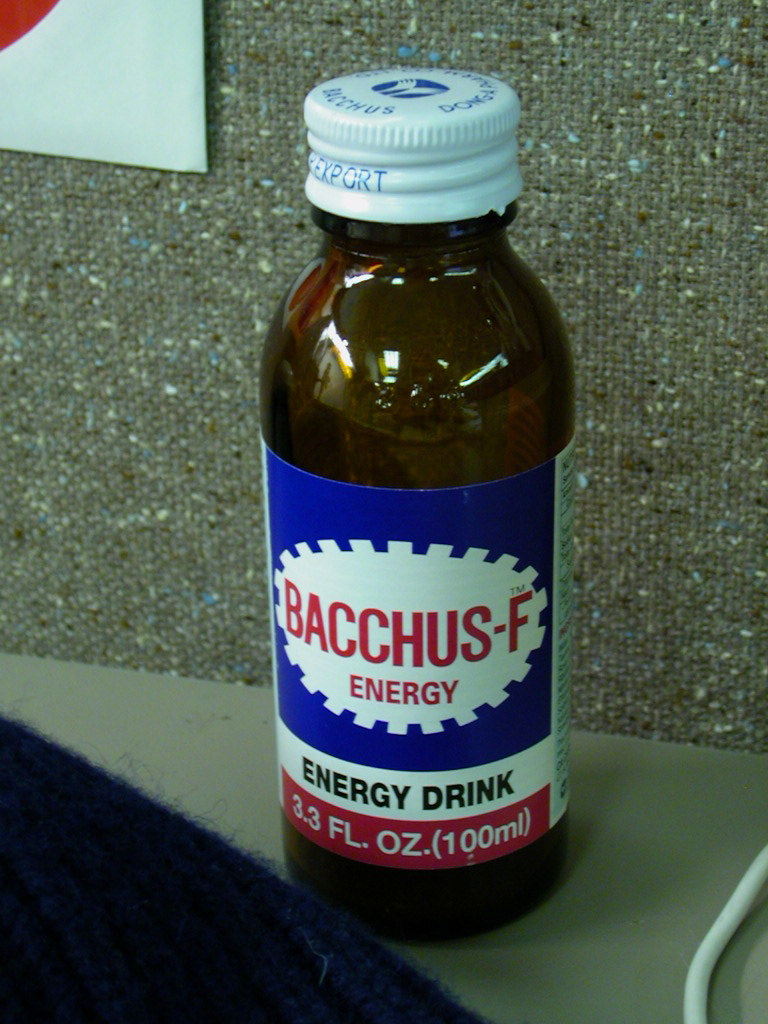This is a color photograph taken in poor lighting, possibly with a filter applied. Dominating the center of the image is a small, dark brown glass bottle of Bacchus-F energy drink. The bottle is capped with a white lid featuring an unreadable blue logo and text that includes the word "export." The front label of the bottle is predominantly blue, displaying a white oval with "BACCHUS-F" in red lettering, followed by the word "energy" in red. Below this, on a white background, "energy drink" is printed in black text, and the bottom of the label features a red strip with "3.3 fl oz (100 mL)" in white. The bottle is placed on a grayish surface, which contains a subtle black triangle towards the bottom left, potentially the edge of the surface. The background appears to be a speckled wall with gray, blue, brown, and beige woven textures. In the top right corner of the image, part of a square tile is visible, and a small red triangle can be seen at the extreme right edge of the photo. There's also a narrow white bar visible in the lower right corner.